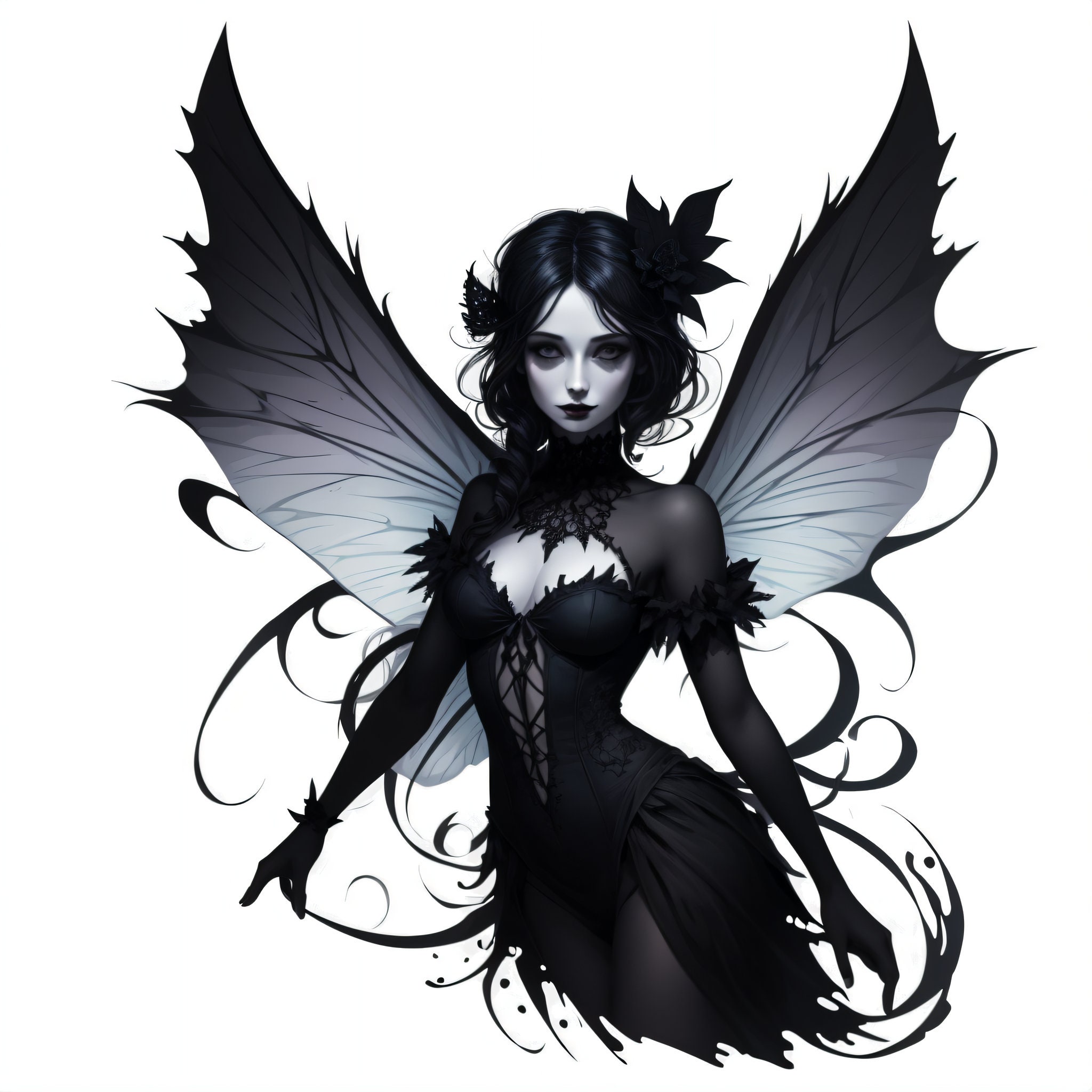The image portrays a digital illustration of a somber, dark fairy-like woman with an anime-inspired style, set against a completely white background. She has extremely pale skin and jet black, wavy hair that just past her chin, adorned with dark, black flowers on either side. Her deeply shadowed eyes and dark eye makeup, along with black lipstick, give her a serious and somewhat melancholic expression. The woman wears an intricate, lacy black dress with a sheer lacy section extending up her neck and down her long sleeves. The bodice of her dress features an open cleavage area, covered by a sheer mesh with string patterns. Her attire is completed with a wispy skirt and dark tights or pantyhose. Adding to her ethereal, yet dark persona, she has large, black, bat-like wings extending from her back, almost reaching above her head, with various black swirls emanating from her figure against the stark white background.